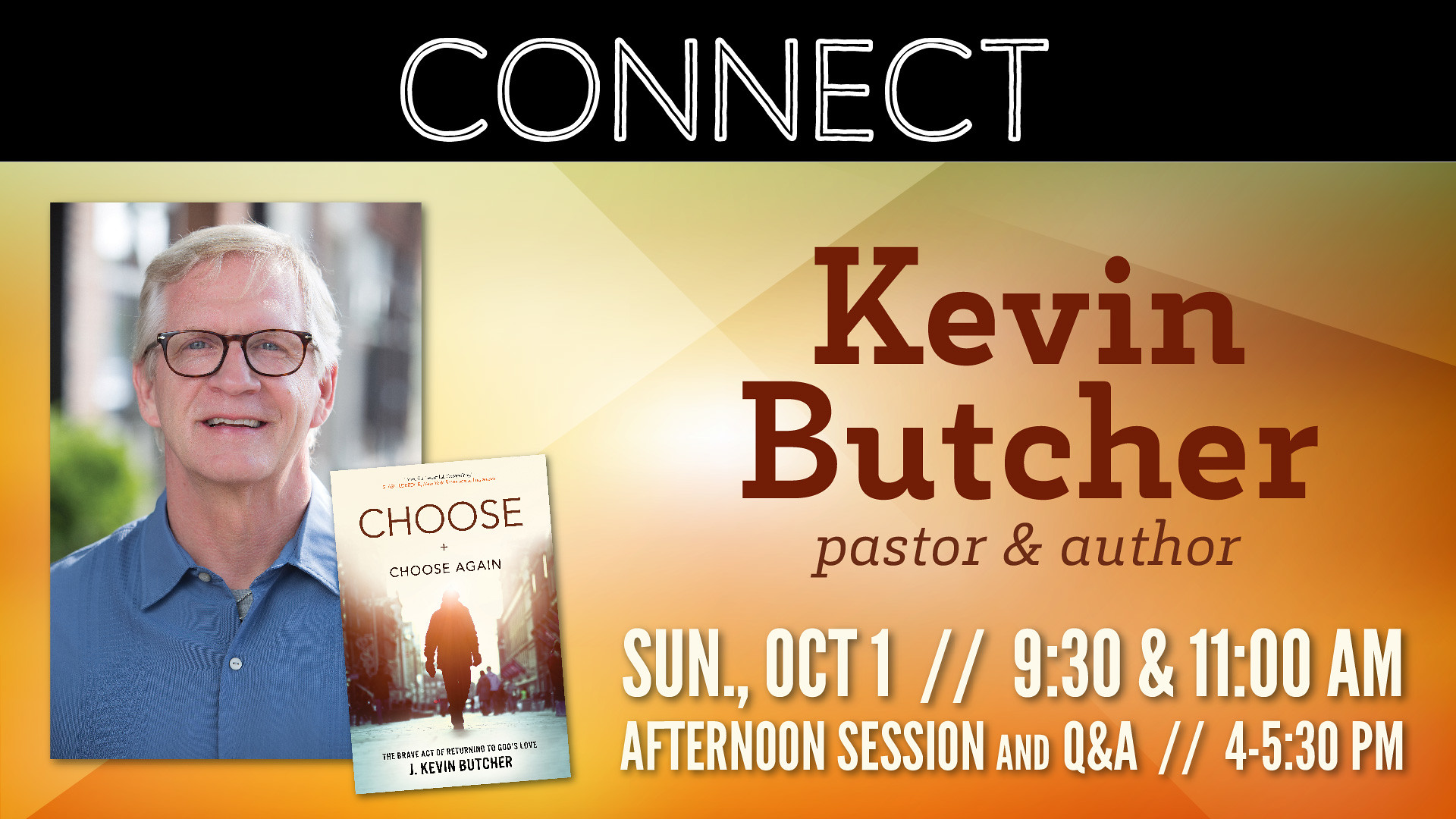The online ad prominently features the word "Connect" in bold white letters at the top against a stark black background. On the left side of the ad, there's an image of an older man with gray hair, wearing black glasses, and smiling warmly. He dons a blue collared shirt. Next to him on the right is the image of a book titled "Choose" with the subtitle "Choose Again." The book is authored by Kevin Butcher. The text in brown letters to the right of the book image reads "Kevin Butcher," followed by "Pastor and Author." In the lower right-hand corner, white letters provide event details: "Sunday, October 1st // 9:30 and 11 a.m.," followed by "Afternoon Session and Q&A // 4 to 5:30 p.m." The ad also features an image related to the book cover, depicting a youthful figure walking toward the light down a city street, emphasizing the book's message of returning to God's love.